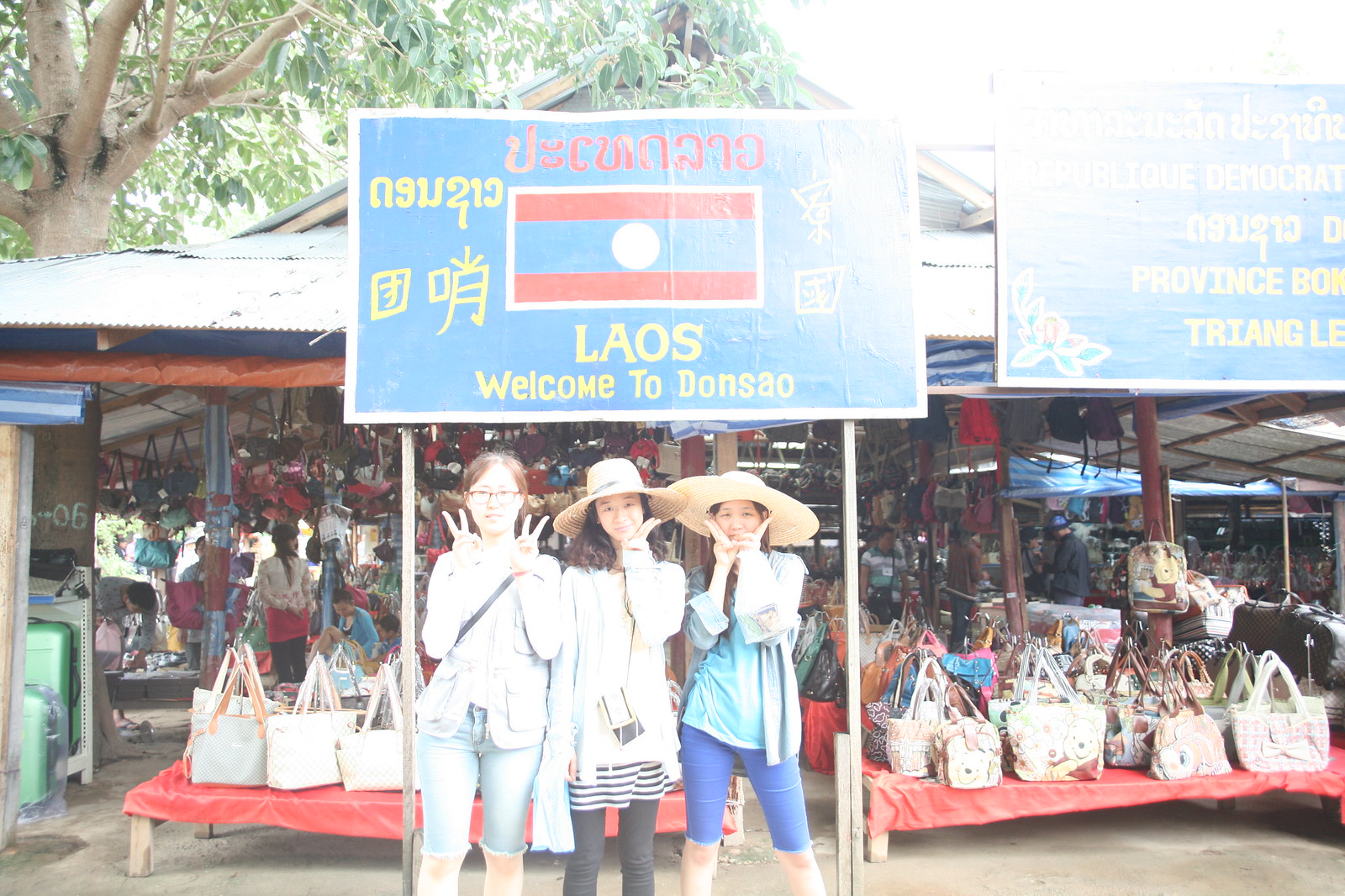In the image, a slightly washed-out and blurry outdoor scene is depicted, featuring three young women standing in front of a shop resembling a market tent. Each of the women is making a peace sign with their fingers—one with both hands, another with one hand under her chin, and the third simply displaying one peace sign. Two of the women are wearing straw hats, and one is wearing glasses. Behind them, there is a low table laden with tote bags and various types of merchandise under the large tent. The shop tent has two prominent, but somewhat unreadable, blue signs with red, white, and blue flag designs. One of the signs appears to say "Layles" with the phrase "welcome to Don's Sale" written underneath in red and yellow letters. A grey sky is visible at the top right of the image, and a tree is on the left side. The overall effect of the photograph is quite bright and has a slightly overexposed quality, contributing to the difficulty in reading some of the text.